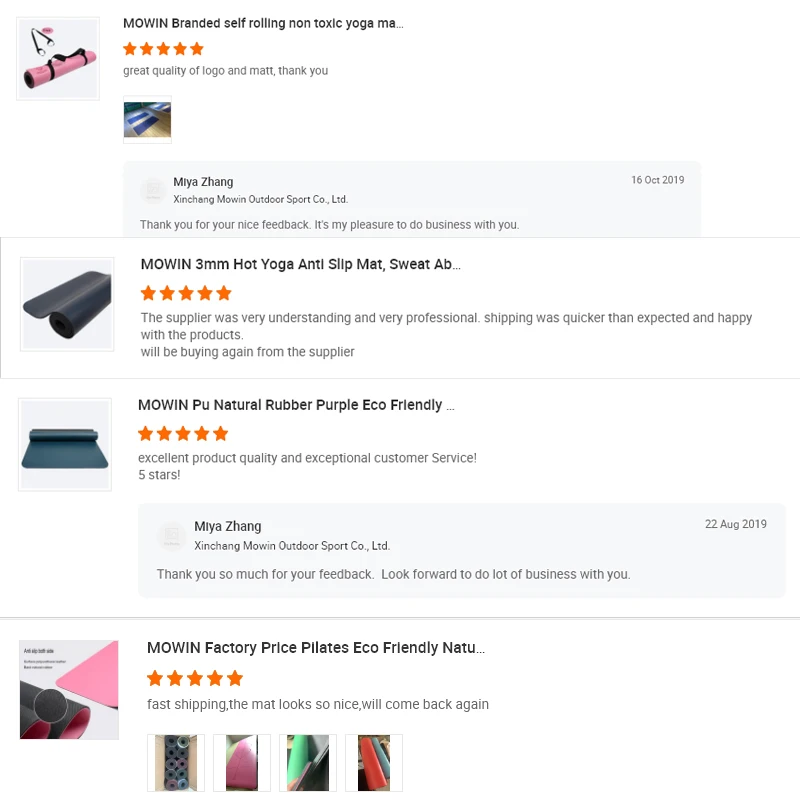This screenshot appears to be taken from an online retailer's website, presumably Amazon. The webpage displays a list of four yoga or workout mats from the brand Moen, as indicated on the left side of the page through product images. Each mat has been rated five stars by customers. 

The page also includes customer reviews and comments from the seller. The seller has responded to the positive feedback with gratitude, saying, "Thank you for your nice feedback. It's my pleasure to do business with you," and "Thank you so much for your feedback. Look forward to doing a lot of business with you." The background of the page is white, contributing to a clean and minimalist design, which emphasizes the product listings and reviews. The overall presentation suggests a well-received product line, reinforcing the brand's positive reputation among consumers.